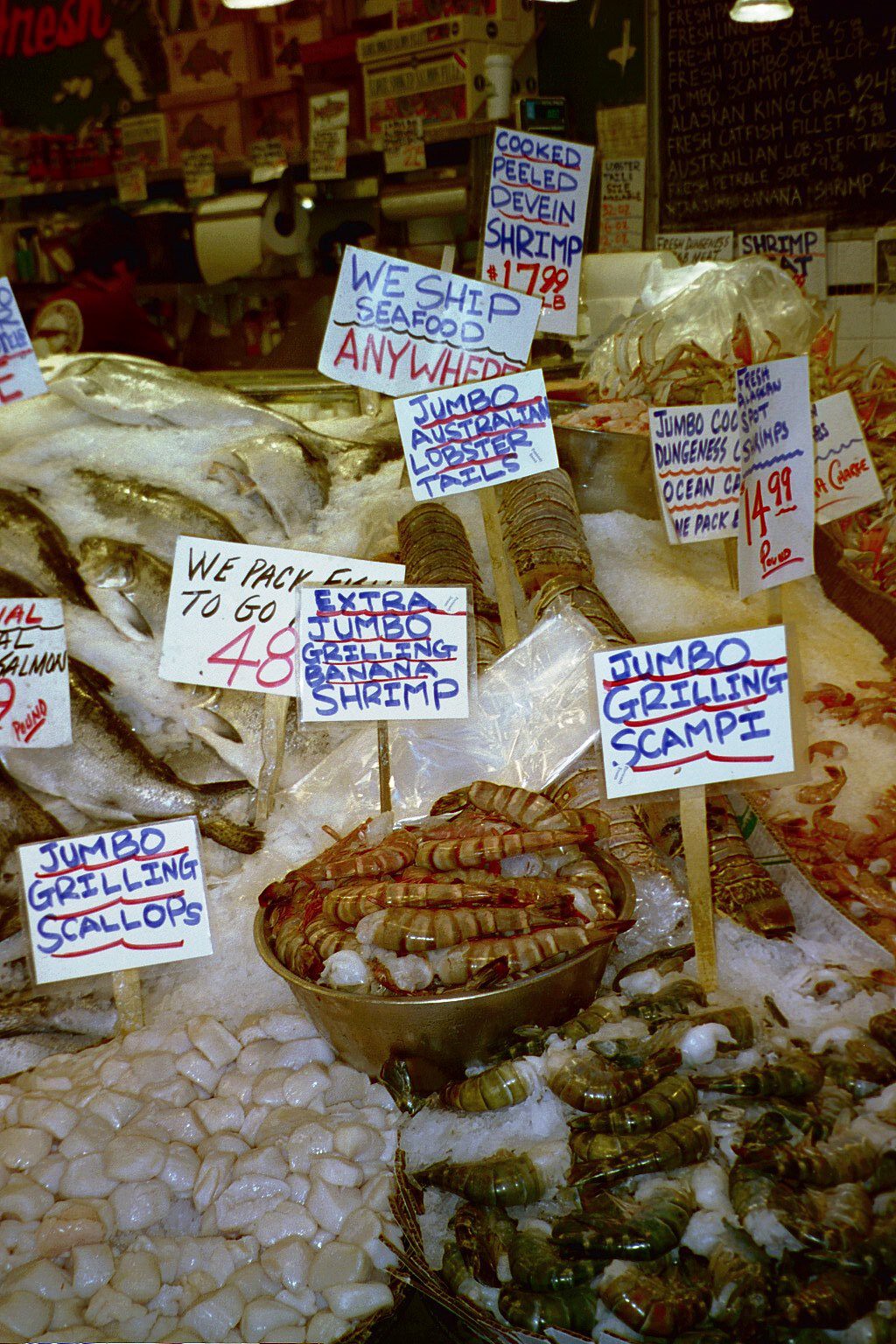This image captures a bustling fish market in Australia, showcasing an array of fresh seafood delicacies meticulously displayed on ice. Prominently featured are jumbo Australian lobster tails, extra jumbo grilling banana shrimp nestled in a pot, jumbo grilling scallops, and jumbo grilling scampi, each variety accompanied by a white sign with blue writing and a red underline. One sign advertises cooked, peeled, deveined shrimp at $17.99 a pound. Additional signs assure customers of convenient services such as "We Pack to Go" and "We Ship Seafood Anywhere." The background reveals a black bulletin board with red writing and a roll of paper towels affixed to the wall, adding to the market's vibrant and well-organized atmosphere.